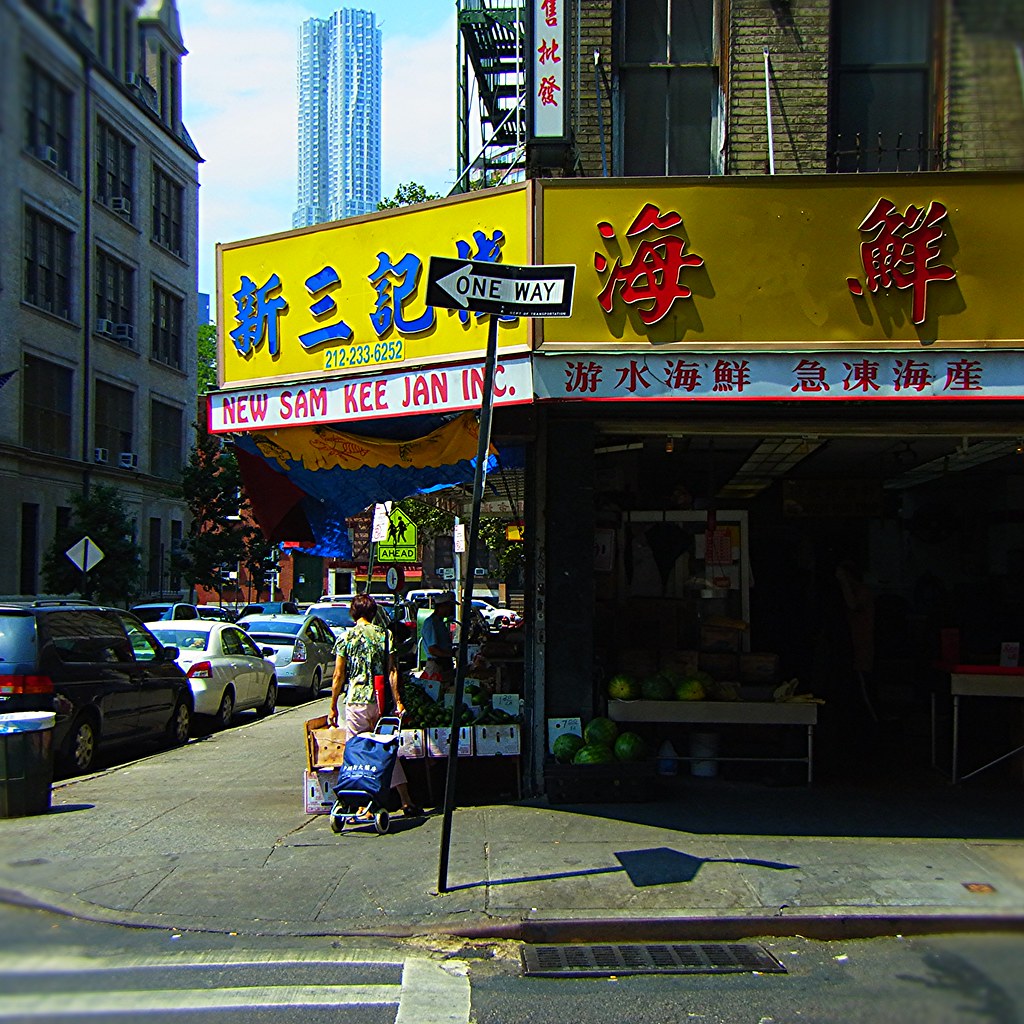This image captures a bustling street corner during the daytime in a city presumed to be in the United States, given the style of street signage. The focal point is a corner market called "New Sam Kee Jan Inc." prominently displayed on a white banner with red lettering below bright yellow banners adorned with blue and red Asian characters. The market features a large canopy extending over the sidewalk, shading tables laden with watermelons in bins. It has an open-air feel, with its front section resembling a patio. A woman is seen examining some of the fruit while pulling a cart, and more tables are visible through a partition to the left. The street slopes slightly downward toward a crosswalk painted on the pavement, where a sewer grate is also visible. There's a tall street sign indicating a one-way street, and in the background, a towering skyscraper rises against a partly cloudy blue sky. Cars are parked along the street, and a building across the road bears a school crossing sign. The scene is lively and detailed, offering a snapshot of urban life at this vibrant street corner.